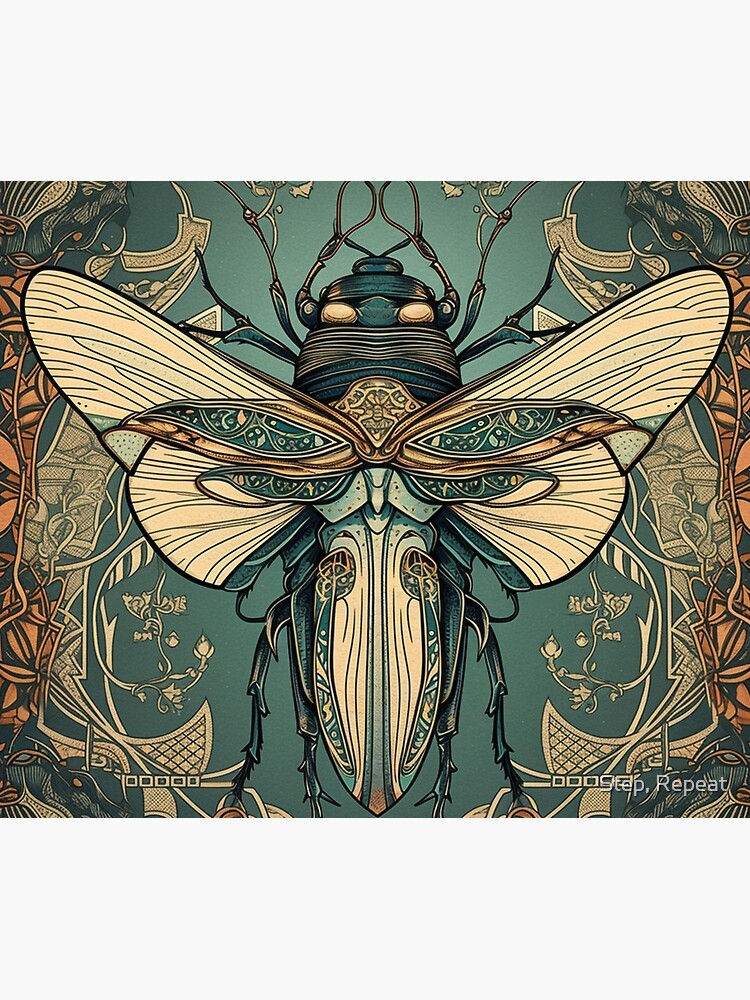This image depicts a stylized artwork of an insect resembling a moth, beetle, or fly, set against a teal background. The insect features beige wings that are multi-layered and curving outward, adorned with intricate gold and teal filigree designs and black lines that extend from the base to the edges of the wings. The insect has several legs extending from its thorax and rear, and tentacle-like pinchers protruding from its face. The artwork is housed within a larger rectangular frame, which contains a more squared inner frame, both adorned with symmetrical, intricately woven shapes in yellow and light orange, reminiscent of leaves. The entire piece is executed in dark colors with prominent greenish, gold, and brown tones. In the bottom right corner, there is text in English that reads "step repeat." The overall design is highly detailed and symmetrical, reflective of the insect and the surrounding motifs.